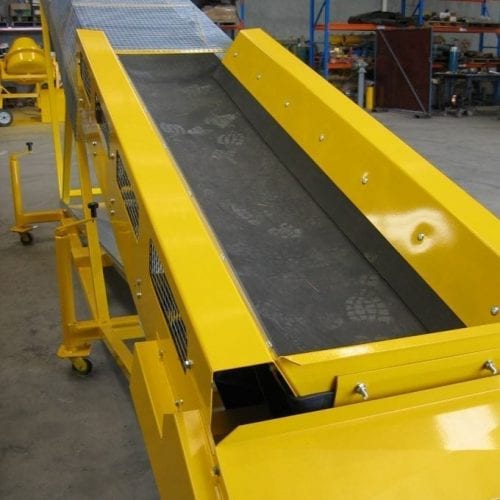In the image, there is a bright yellow industrial machine centrally positioned within what appears to be a warehouse or industrial setting. The large, rectangular machine extends diagonally upwards, resembling a conveyor with a distinctive black belt section running through its middle. The black belt section bears footprint impressions, indicating use. The machine is equipped with small black wheels, two of which are visible on the left side, suggesting it is mobile.

In the background towards the upper part of the image, there are several carts with various objects placed on them. Additionally, shelves filled with miscellaneous items are visible in the upper right corner, contributing to the industrial ambiance. A secondary bright yellow machine can be seen in the upper left corner, alongside what appears to be a concrete mixer on the back wall. The floor around the central machine is mostly an open, wide space, and the overall color palette includes shades of gray, yellow, black, silver, red, and blue. There are no people present in the image, and no text or labels are visible.